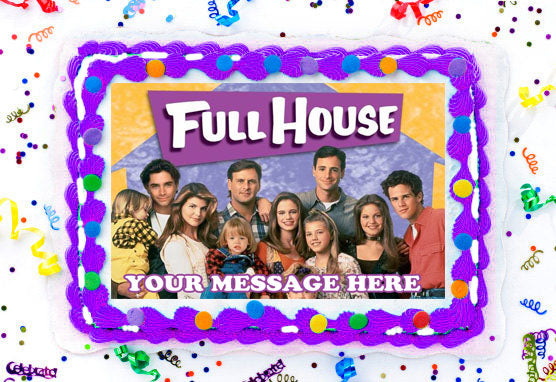This is a horizontally rectangular image resembling a product advertisement for a customizable item. The image features a pristine white background adorned with vibrant, scattered dots of blue, green, orange, and purple, reminiscent of confetti or festive ribbons. At the center, a highly stylized cake decorated with white frosting and a double layer of purple icing, accented by circular colored elements, possibly candy or chocolate chips, catches the eye. The focal point within the cake is a trapezoid-shaped purple box with the iconic "Full House" logo in bold white letters with a black shadow. Below this, a nostalgic photo of the youthful cast of the Full House TV show prominently displays, bringing a touch of friendly familiarity. The space beneath the cast photo is reserved for customizable text, where the message "Your message here" appears in a white font outlined in purple, suggesting that buyers can personalize this area to fit any occasion. This image bridges the simplicity of a greeting card with the celebratory charm of a customized cake, making it a versatile product for gifting or personal keepsakes.